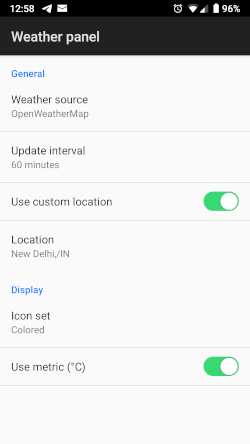Screenshot of a cell phone screen with a black background at the very top. The left side shows "12:58," followed by a mail icon. To the right, there are icons for an alarm clock, Wi-Fi signal, and cell signal, with a fully charged white battery icon displaying "96%". On the left side, in gray text, it says "Weather Panel".

Below this, on a white background, the top section has "General" in blue text. The subsequent text, in black, reads "Weather Source" and below that, in gray, "OpenWeatherMap". The next line in black reads "Update Interval", followed by "60 minutes" in gray.

Further down, in black, it reads "Use Custom Location" with a green slider indicating it's turned on. The location is specified as "New Delhi/IN" (assumed to be New Delhi, India).

Next, in blue text, it says "Display". Below it, in black, it says "Icon Set" and in gray, "Colored" (spelled in American English). At the bottom, in black text, it says "Use Metric (°C)" with a gray toggle switch beside it, turned on.